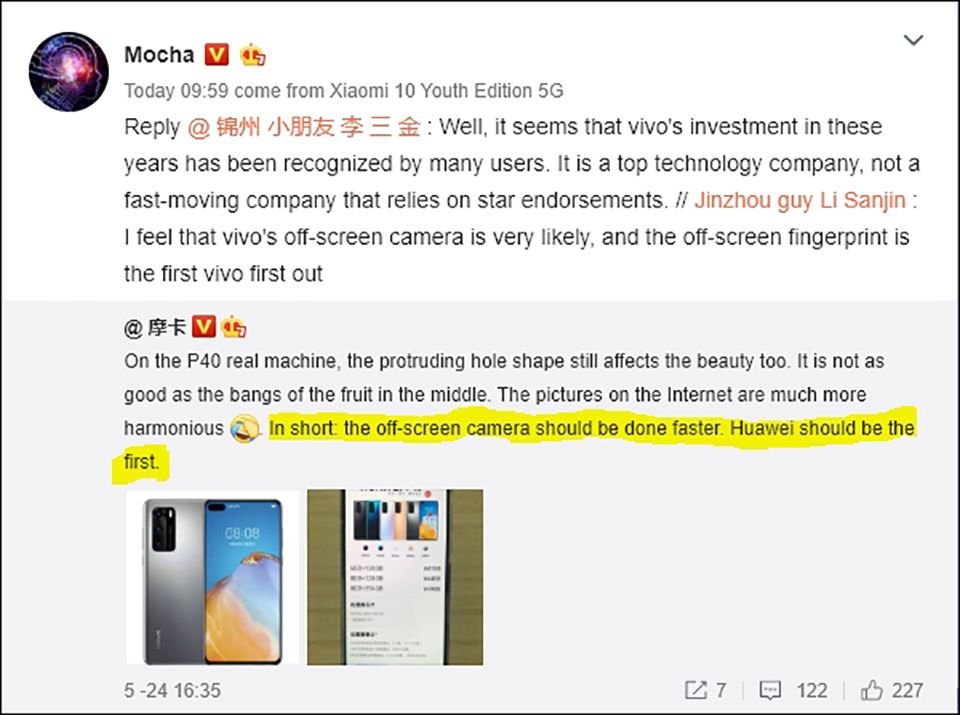Screenshot of an online platform showing a discussion about Vivo's technological advancements. The username “Mocha” is displayed in the upper left-hand corner. Mocha has replied to a comment, stating that Vivo’s substantial investments over the years have garnered recognition from many users. They emphasize that Vivo is a top technology company, known for innovation rather than relying solely on star endorsements. Mocha expresses optimism about Vivo's off-screen camera technology and in-screen fingerprint sensors, suggesting Vivo might be the first to release these features. They are responding to another user who mentioned that the protruding hole on the Huawei P40 model's screen impacts its aesthetics negatively, comparing it unfavorably to more centrally aligned designs seen in online images. The user hopes for quicker development of off-screen camera technology, indicating that Huawei should lead this innovation. Below these comments are two images showcasing a mobile device, hinting at the ongoing discussion being centered around mobile phone design and technology.